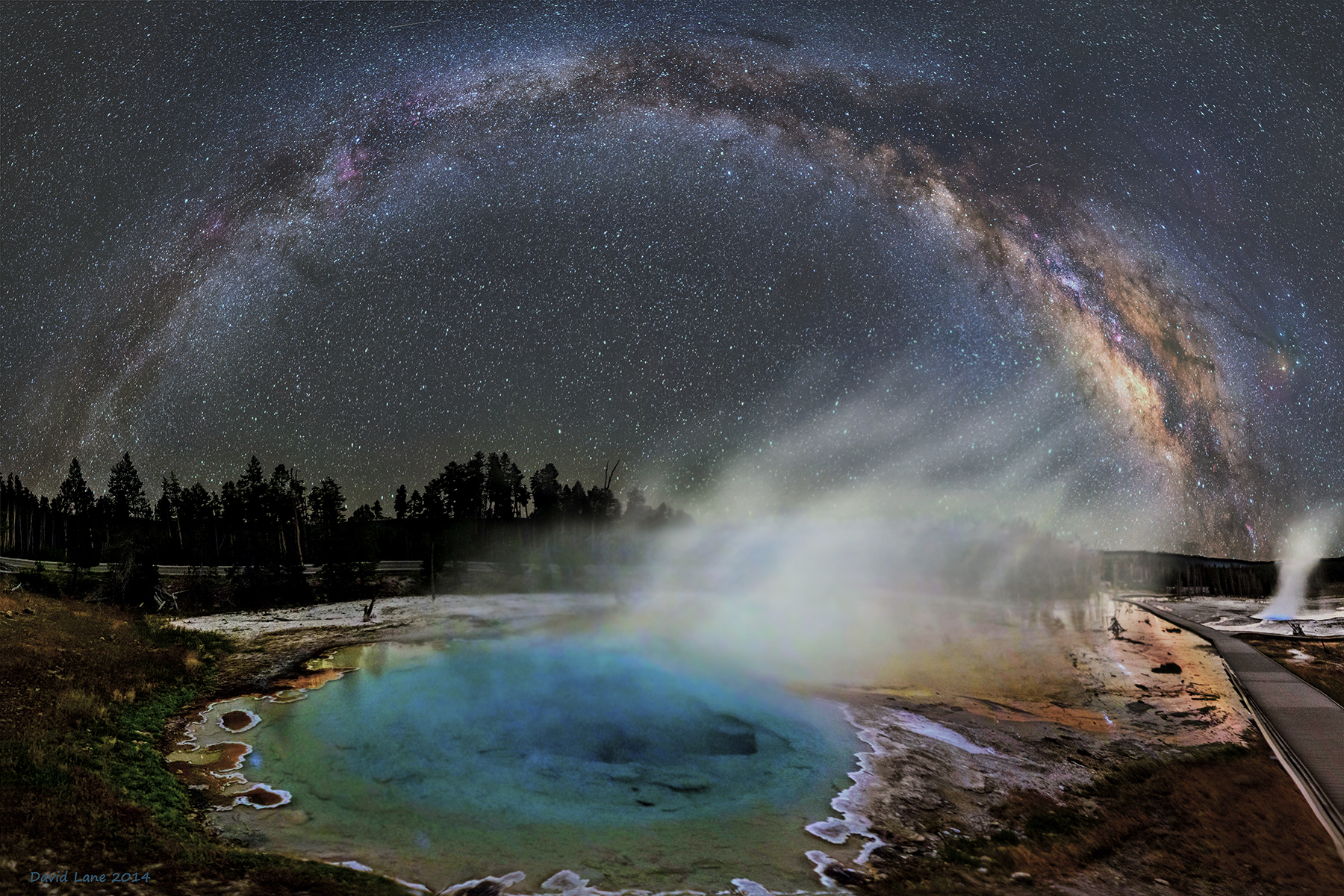This image, likely computer-generated, depicts a striking night scene. A dark gray sky, filled with an abundance of stars and resembling the Milky Way, forms the backdrop. This sky features a notable rainbow-shaped arc with delicate lavender highlights and darker blue and brown tints on its underside. It's punctuated with tiny white specks, giving the illusion of a galaxy.

In the foreground, a small, circular thermal pool takes center stage. The pool transitions from light yellow around its edges to a clear, deep blue at its center, which appears to house a dark hole or submerged rocks. The edges of the pool are outlined with white salt deposits and possibly sand or dirt. Mist and steam rise from the water, particularly on the right-hand side, where a misty spray ascends towards the upper right corner of the image. Surrounding this pool, to the left, you can see dark gravel and rocks, while green and brown grass appears at the very bottom of the image.

A wooden boardwalk extends just beyond the pool's perimeter on the right, leading to additional smaller pools emitting steam. These pools, surrounded by white sulfur or salt-like deposits, contribute to the otherworldly ambiance. Behind this scene, the terrain slopes slightly upwards, displaying brown and red hues.

In the distance, there is a silhouetted tree line comprising both deciduous and fir trees with visible foliage, rendered in dark greens and blacks. Amidst this setting, on the right, a smaller lithe geyser spews white frost into the air, adding to the surreal quality of the landscape.

This detailed composition captures the tranquility and mystique of a thermal landscape under a mesmerizing night sky, reminiscent of Yellowstone National Park.